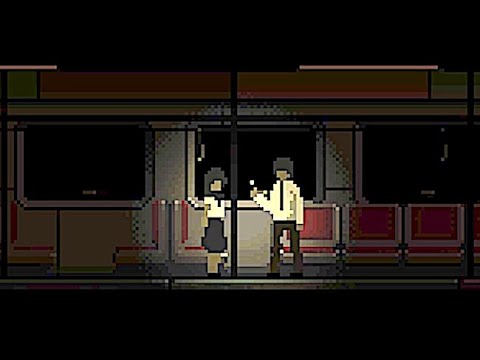The image appears to be pixelated artwork resembling an old-timey video game from the 80s or 90s. It depicts the dimly lit interior of a subway car, with the only illuminated figures being two characters standing in front of a central pole. The woman on the left has brown hair and is dressed in a white short-sleeved shirt and a black skirt, while the man on the right wears a white shirt with a black tie, black pants, and has curly black hair, holding an unspecified object in his hand. The subway car features red seats and windows, with yellow and white walls that contrast against a pitch-black background, giving the scene a dissected, inside view as though it’s dark all around except for the spotlight on the characters. The art is static and simplistic, with minimalistic color use typical of classic video games.